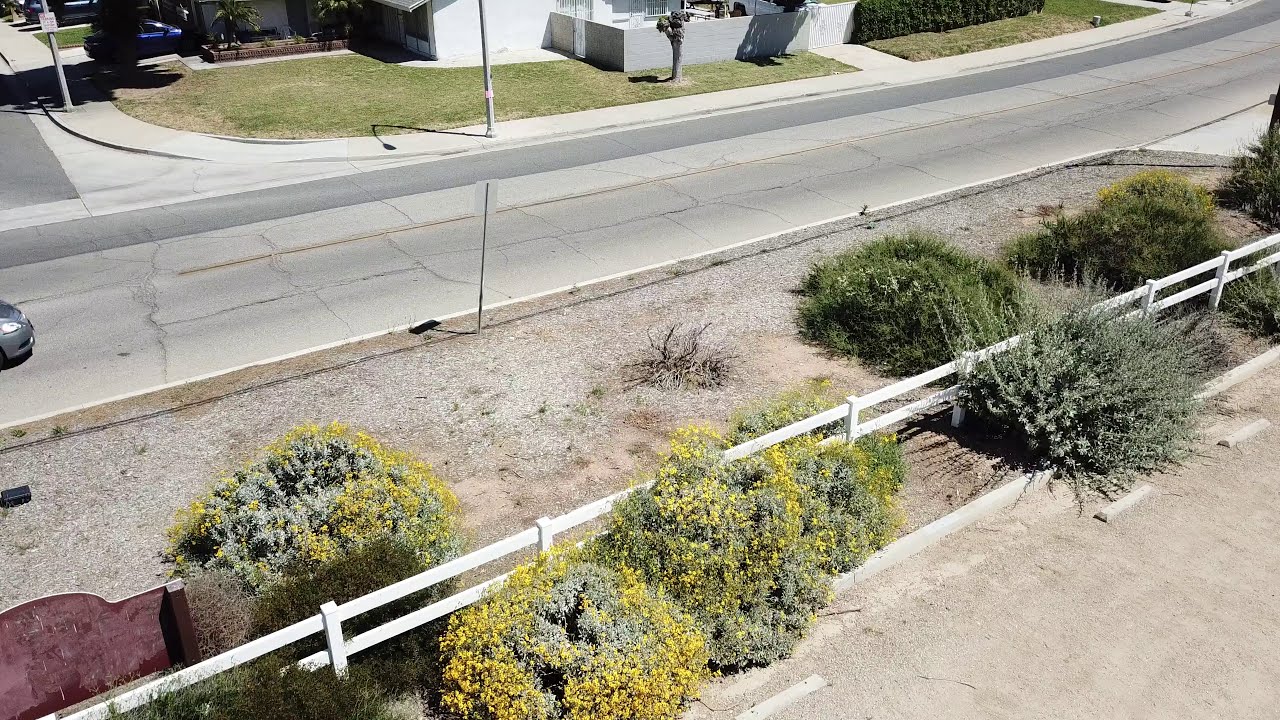The image depicts a serene corner of two intersecting roadways, with the scene extending off into the right-hand distance. A silver car is just making its way into the frame from the left. The foreground is dominated by a sign whose text faces away from the viewer. Surrounding the roadway, there is a patch of land adorned with a variety of bushes, including some that bear tiny yellow flowers. Prominently, a white picket fence runs diagonally from the lower left to the right edge of the image, partially enclosing an area that seems to be a mix of dirt and greenery. Behind the fence and bushes, a side panel of a house with surrounding green grass is visible, suggesting a residential neighborhood. A sidewalk and parking spaces appear just beyond the fence. The scene has a touch of wilderness, accentuated by the mix of grayish-green shrubbery and the rustic, dirt-covered areas.